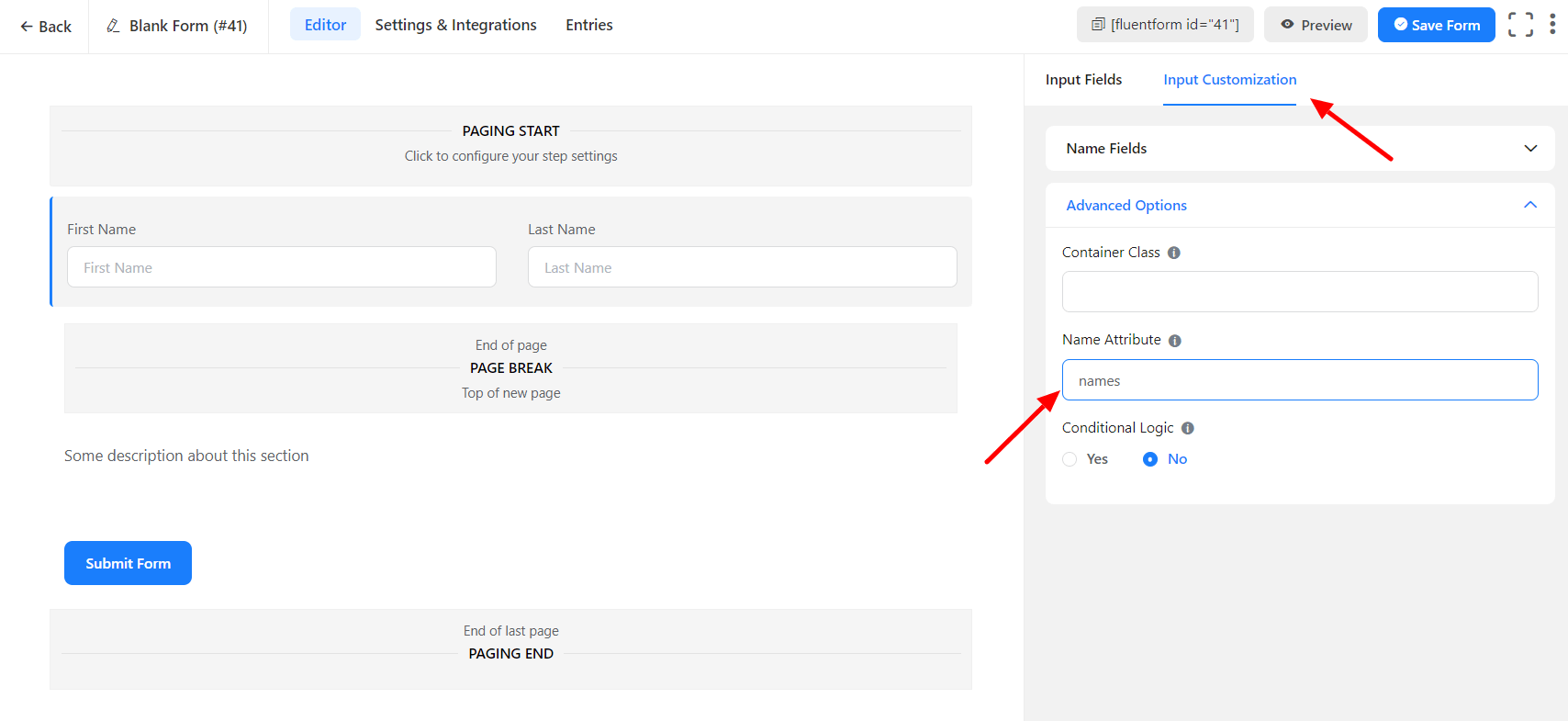The image showcases two screenshots side by side, each capturing different segments of a form-building interface.

On the left screenshot:

- At the top, there is a back arrow icon.
- Directly below the back arrow, there's a blank form area.
- To the right of the blank form area, there are three tabs labeled: "Editor," "Settings and Integrations," and "Entries," with the "Editor" tab currently selected.
- Below the tab menu, there is text that reads "Page Start," followed by the prompt "Click to configure your step settings."
- Further below, there are input fields for "First Name" and "Last Name."
- Continuing down, it mentions "End of Page," "Page Break," and "Top of New Page."
- Below these sections, there's an input field labeled "Some description about the section."
- At the bottom of this screenshot, there is a blue "Submit Form" button.

On the right screenshot:

- The interface prominently displays three tabs at the top: "Preview," "Fluent Form ID," and "Save Form," with the "Save Form" tab currently selected.
- Within the selected tab, the "Input Customization" section is visible.
- There is a text input field labeled "Name Attribute."

The image collectively captures the detailed layout and options available in a form-building interface, illustrating various stages and components of customizing and saving a form.